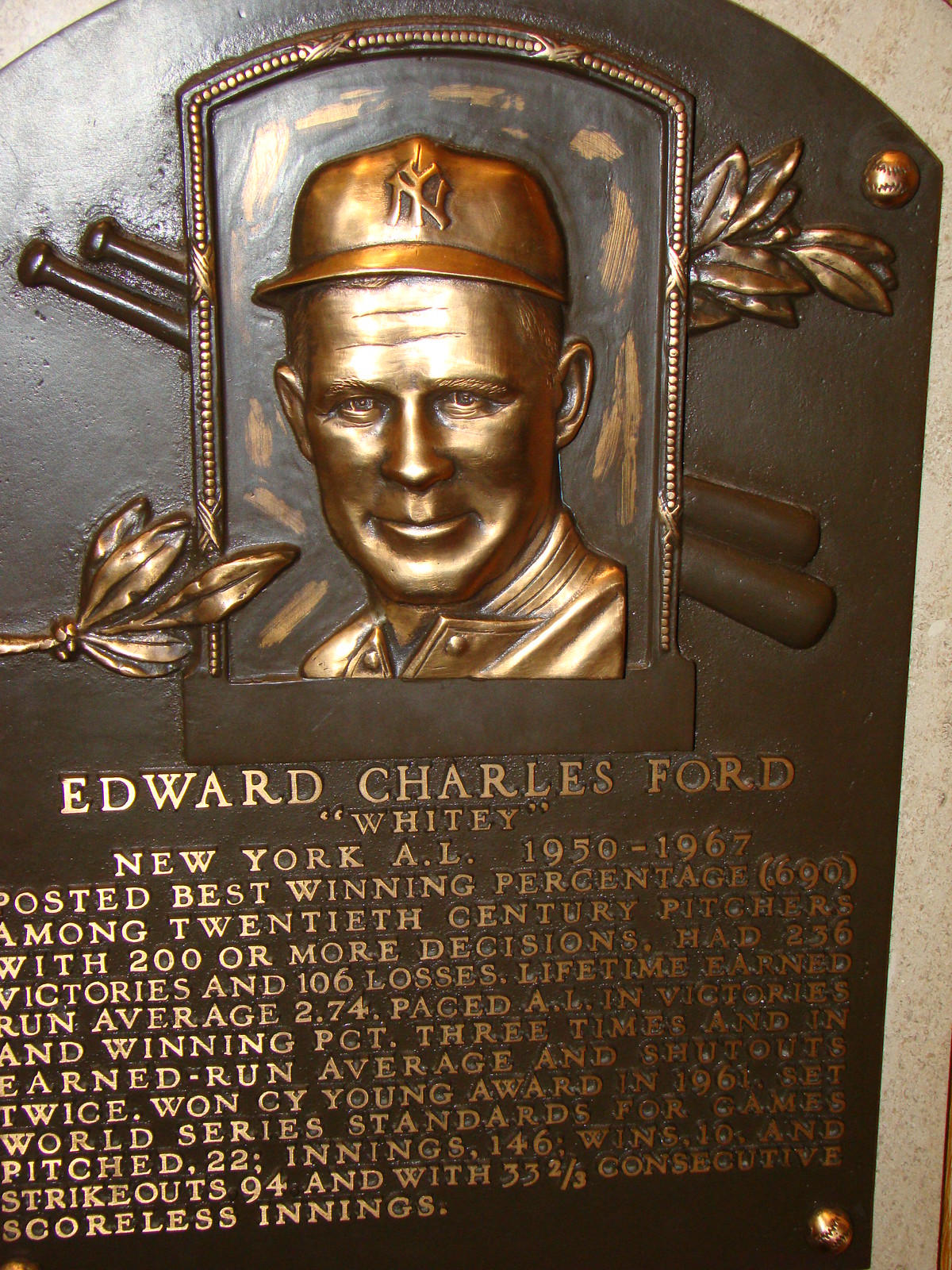This photograph showcases the Hall of Fame plaque for Edward Charles "Whitey" Ford, prominently displayed in the monument section of Yankee Stadium. At the top of this bronze plaque, there is a detailed relief image of Ford, adorned with a New York Yankees cap, and surrounded by a goldish wreath. Flanking the image are two baseball bats. The plaque is rich in detail, with leaves extending from the left and right. Underneath Ford's image, his official name "Edward Charles Ford" appears, along with the nickname "Whitey." Below this, the inscription reads "New York A.L. 1950-1967." The plaque provides a wealth of information about Ford's illustrious career, highlighting his best winning percentage among 20th-century pitchers with over 200 decisions and noting his Cy Young Awards and World Series accomplishments. The bronze plaque sits against a brown background, itself mounted on a beige concrete wall, lending a stately and reverent air to this tribute.